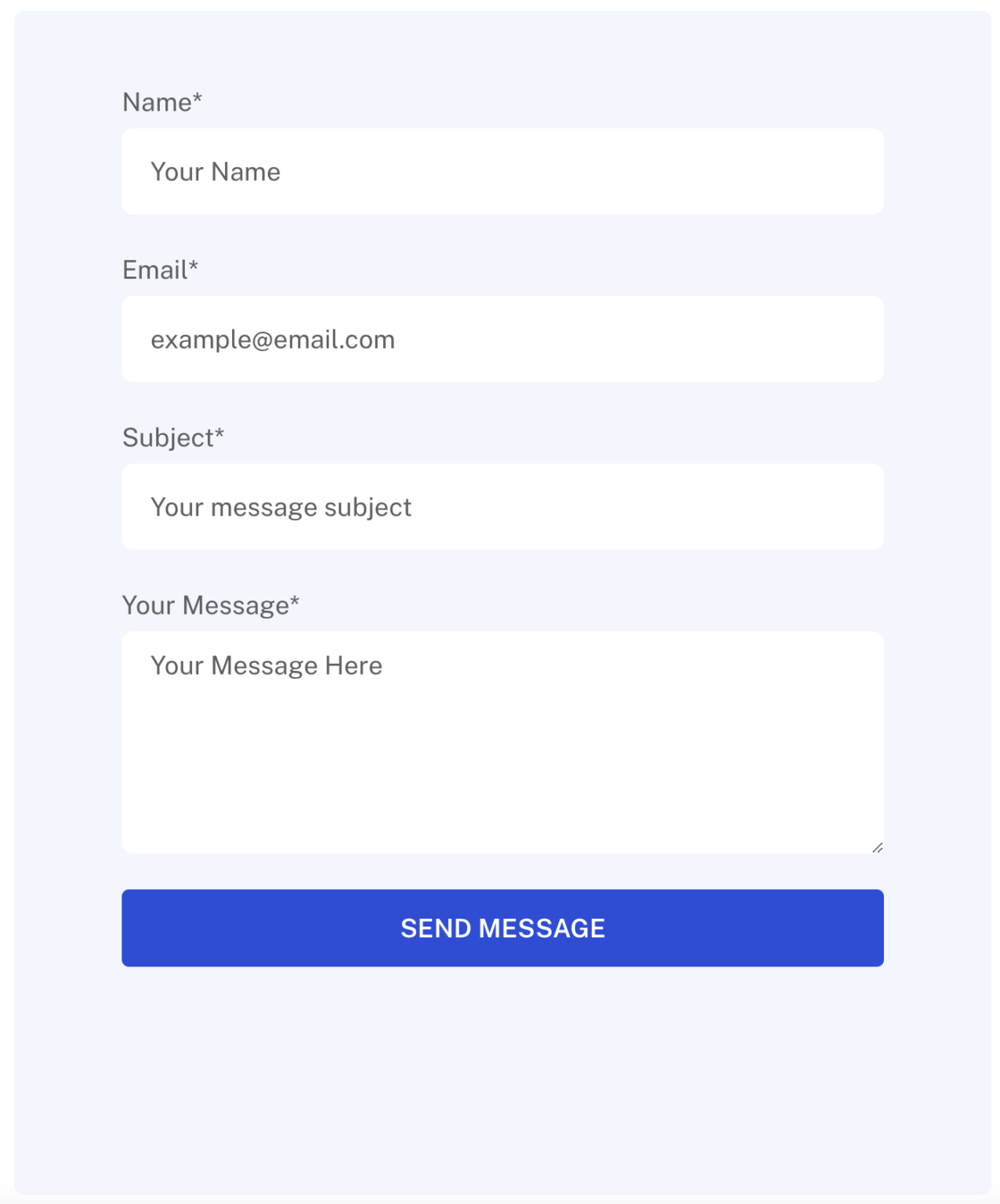The image is a simple, vertically-oriented screenshot of a message form, set against a white background. The form itself is encased in a very pale blue, almost grayish, rectangle. 

At the top of the form, the label "Name*" appears in black text, indicating a required field. Beneath this label is a white, long, rectangular input field with placeholder text "Your Name," with the first letters of "Your" and "Name" capitalized.

The next field down is labeled "Email*" in black text, also signifying a mandatory entry. The accompanying input field contains the placeholder text "example@email.com" in lowercase letters.

Further down, the form presents the label "Subject*," followed by a white input field that reads "Your Message Subject," again with the first letters of each word capitalized.

The final field is labeled "Your Message*" in black text, with a larger input area beneath it. This field contains the placeholder text "Your Message Here," where each word's first letter is capitalized.

At the bottom of the form, there is a long blue button with the text "Send Message."

Overall, the form is designed for a user to input their name, email, subject, and message before submitting via the blue button.